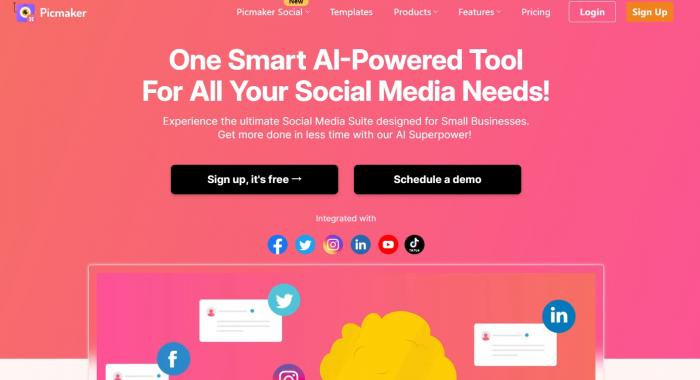The splash page for Pickmaker, a business specializing in social media management tools, features a sleek and user-friendly design. Positioned in the upper left corner is the company's logo, adjacent to the brand name "Pickmaker" in crisp white letters. The entire background is a vibrant pink, lending a lively and modern feel to the interface.

At the top of the page, a navigation bar presents the following sections: Pickmaker Social, Templates, Products, Features, Pricing, Login, and Signup. The "Pickmaker Social," "Products," and "Features" tabs are each marked with a small pink downward arrow, indicating the presence of drop-down menus. The "Login" button is outlined in light pink, while the "Signup" button stands out with an orange background and white text, ensuring it's easily noticeable.

The main headline captures attention with its bold white font, stating, "One smart AI-powered tool for all your social media needs." Beneath this, a subheading in smaller white letters entices users with, "Experience the ultimate social media suite designed for small businesses. Get more done in less time with our AI superpower."

Two prominent black horizontal rectangular buttons offer clear calls to action. The left button reads, "Sign up, it's free," in white text, encouraging immediate engagement, while the right button states, "Schedule a demo," also in white text, inviting users to learn more about the product.

Further down, the page highlights integration with major social media platforms through recognizable icons for Facebook, Twitter (now known as X), Instagram, Indeed, YouTube, and TikTok. Below these icons, additional rectangles simulate social media information from Facebook, Twitter, Instagram, and Indeed, offering a visual representation but no actual data.

Overall, the splash page effectively combines a vibrant visual design with clear, inviting messaging to encourage new users to sign up and explore Pickmaker's offerings.